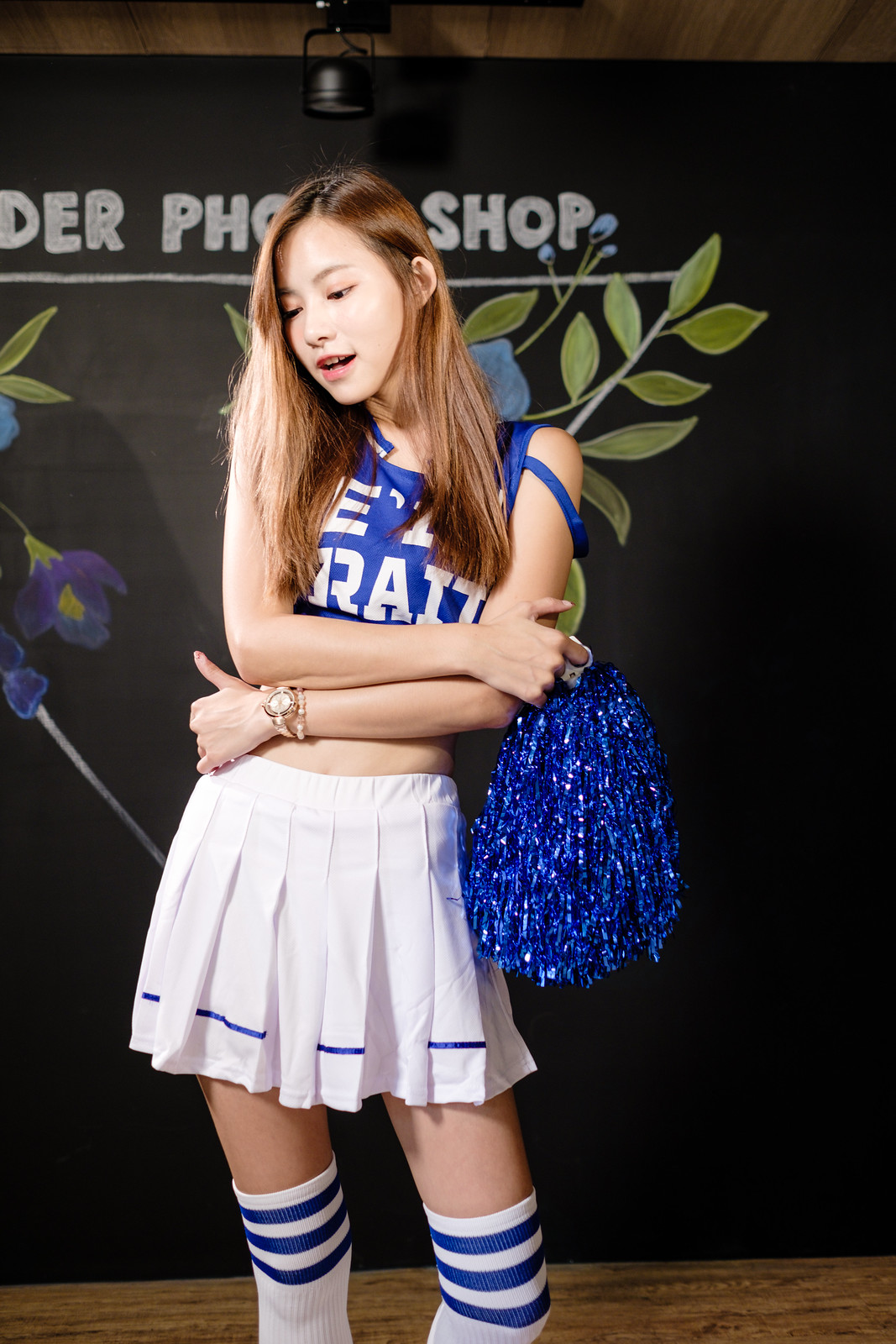The image features a young Asian female cheerleader with distinct Asian facial features, accentuated by her long, dyed light brown hair. She is dressed in a partially exposed cheerleading uniform consisting of a royal blue top with indistinct white writing, and a white pleated mini skirt adorned with a blue stripe at the hem. Her outfit is complemented by white knee-high socks featuring three blue bands near the top. She sports a bracelet and a wristwatch on her left wrist, which is crossed over her midriff, and in her other hand, she holds a blue glittery pom-pom. The background reveals a black, chalkboard-like banner with floral drawings and the fragmented word "SHOP" partially obscured by her head. The cheerleader is looking downward to her right, appearing to be mid-sentence with her mouth slightly open.